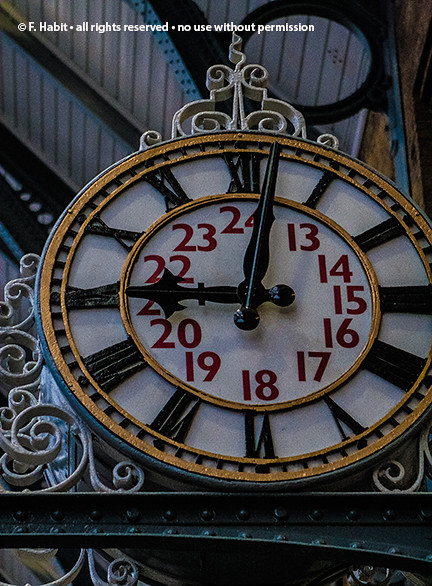This detailed full-color photograph captures an ornate outdoor clock positioned against a backdrop of a building supported by brown metal braces. The clock, encased in a black circular border, sits atop a green metallic girder, which may create an optical illusion suggesting its position. Adorned with white ornamental spirals, the clock face features both Roman numerals (I to XII) on the outer ring and red Arabic numerals (13 to 24) within, allowing it to display time in both standard and military formats. The hour hand points to 21, indicating 9 PM, and the minute hand is just past 24. The structure above the clock includes a white roof supported by brown girders. Notably, at the top left of the image, there is a small inscription: "f.habit. All rights reserved. No use without permission."